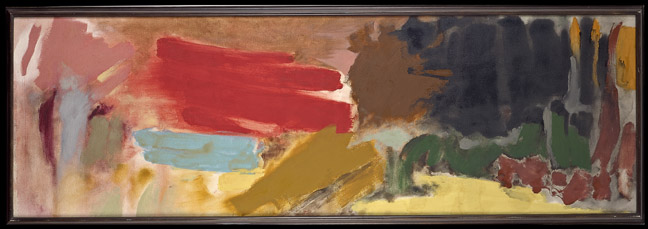The image shows an abstract painting, already framed in a 1-inch thick black frame. The painting is rectangular, longer than it is tall, and features an array of colors including tan, red, sky blue, various shades of green, clayish brown, black, dark green, orange, pink, yellow, and white. The colors are applied in a random, expressive manner with heavy textured paint strokes. The shapes appear to be created by finger or brush movements, giving the artwork a dynamic, back-and-forth pattern. The painting doesn't depict any specific image, lending it an open to interpretation vibe, possibly hinting at an animal or a forest abstractly.